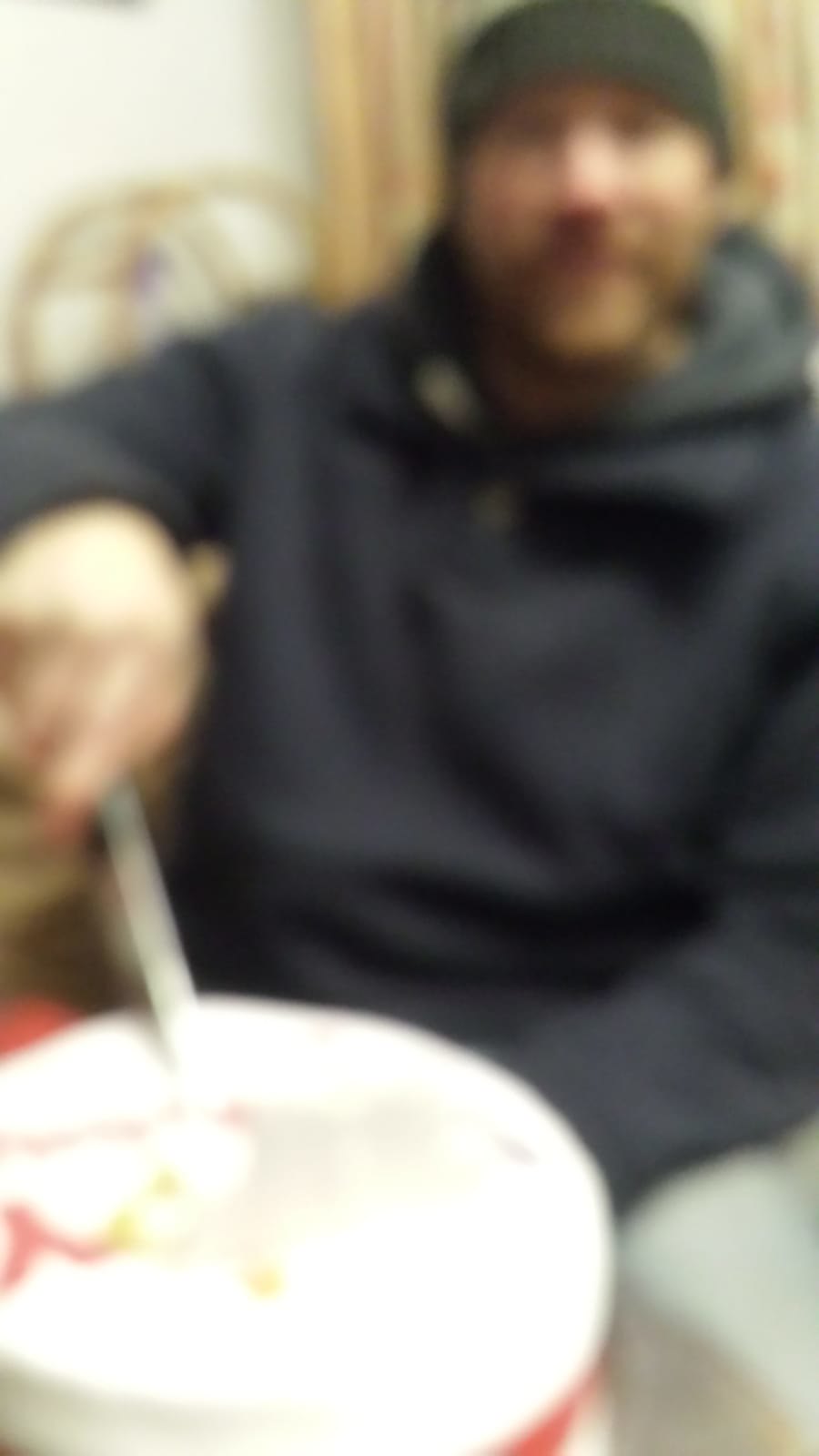The image depicts a blurry scene of a man in the background, identifiable by his black cap, dark gray hoodie, and short brown beard, sitting on a gray couch. He is holding a knife in his right hand and appears to be cutting into a cake in front of him. The cake features white icing adorned with red and yellow decorations, and it rests on a red table. The poor focus of the photo makes the details around the man particularly indistinct, but the vibrant red table and the cake's colorful embellishments stand out clearly amidst the blur.